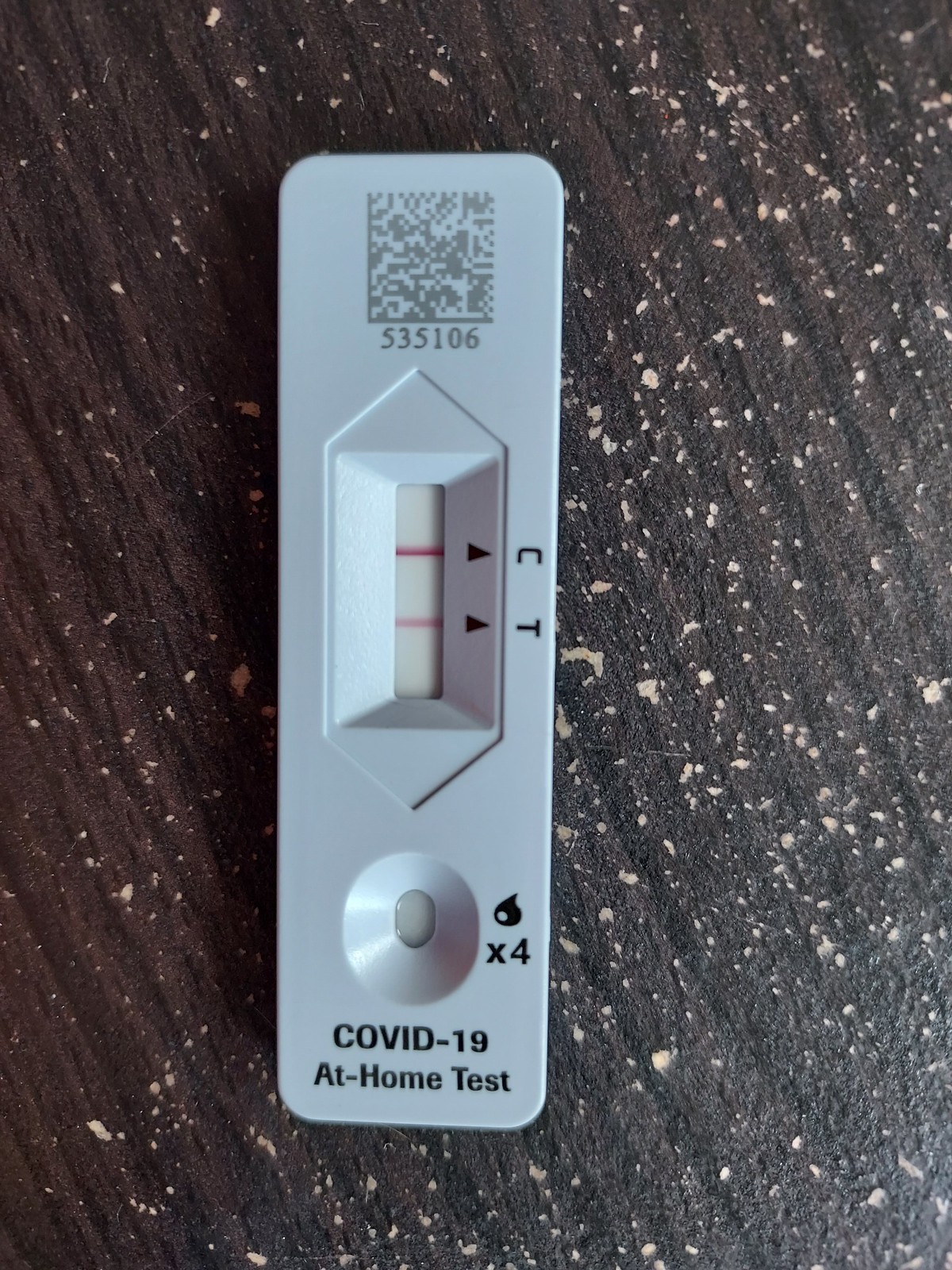The image features a COVID-19 at-home test kit made of light gray plastic, resting on a surface that appears to be either a wooden table or fabric, characterized by dark brown color with diagonal lines or grain running from the top left to the bottom right. The surface also shows lighter tan or white splatters, accentuating its texture. 

The bottom portion of the test kit prominently displays the label "COVID-19 At Home Test." Above this, there's a small reservoir marked with "X4" and accompanied by a stylized droplet symbol, indicating that four drops of the sample should be deposited there. Directly above the reservoir is the readout area, featuring a rectangular window flanked by two diamond shapes at its top. 

Inside the readout window, a dark red control line (C) is visible, with a small black triangle pointing towards the letter "C." A lighter red test line (T) is also present, marked by a black arrow pointing towards the letter "T." This indicates that the test result is positive for COVID-19.

At the top of the test kit, a QR code is visible, followed by the numerical sequence "535106."